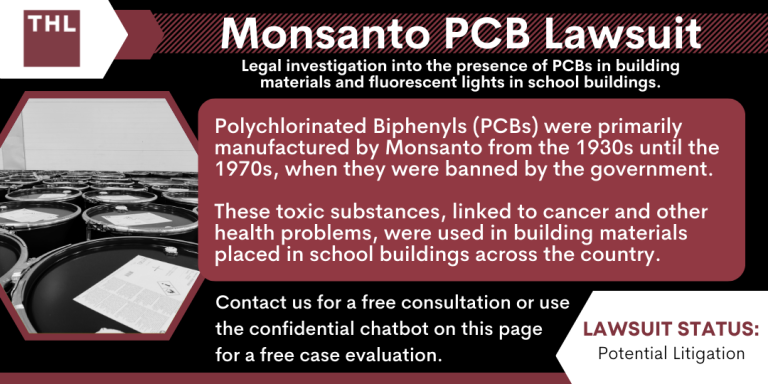The image is an informational advertisement for a Monsanto PCB lawsuit, featuring a deep burgundy brown background with a maroon banner at the top reading "Monsanto PCB Lawsuit" in large white text. Directly below this, a white-on-brown text states: "Legal investigation into the presence of PCBs in building materials and fluorescent lights in school buildings." A smaller banner in a lighter burgundy details: "Polychlorinated Biphenyls (PCBs) were primarily manufactured by Monsanto from the 1930s until the 1970s, when they were banned by the government. These toxic substances, linked to cancer and other health problems, were used in building materials placed in school buildings across the country." 

Towards the bottom, two sections of text include: "Contact us for a free consultation or use the confidential chatbot on this page for a free case evaluation" on a black banner, and "Lawsuit Status: Potential Litigation" on a white background. The top left corner features a THL logo inside a maroon square with a white arrow. The left side of the image has a narrow strip depicting industrial oil drums or barrels that are sealed shut with pieces of white paper on top.